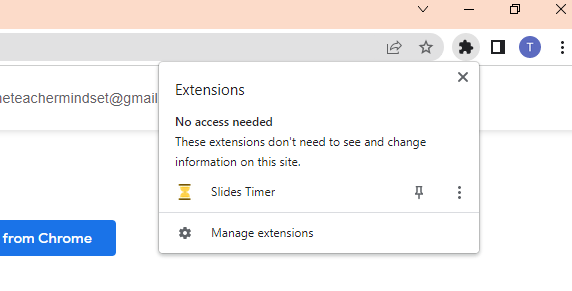The image illustrates a detailed interface of a browser extension toolbar. At the top, a prominent red bar is visible, displaying a downward arrow, a negative sign, squares, and an X icon. Adjacent to the red bar, there's a gray circle followed by an alignment of varied icons including an arrow, a star, and a puzzle piece. 

The words "big T..." are noticeable, followed by the title "teacher, mindset" with an associated email address formatted as "@T-Mail". The interface further includes options labeled as "extensions," though it indicates "not extended," suggesting inactive or minimized extensions. Additional icons resembling an hourglass, a slice timer, and a pen are also present.

At the bottom of the interface, there's a mention "from Chrome," with a blue accent, hinting at it being a Chrome extension. The backdrop of the image is notably light with gray lines, creating a minimalistic and clean visual presentation. The overall setup appears to be a part of a website or application intended to manage or customize browser extensions, likely tailored for educational purposes based on the "teacher, mindset" reference.